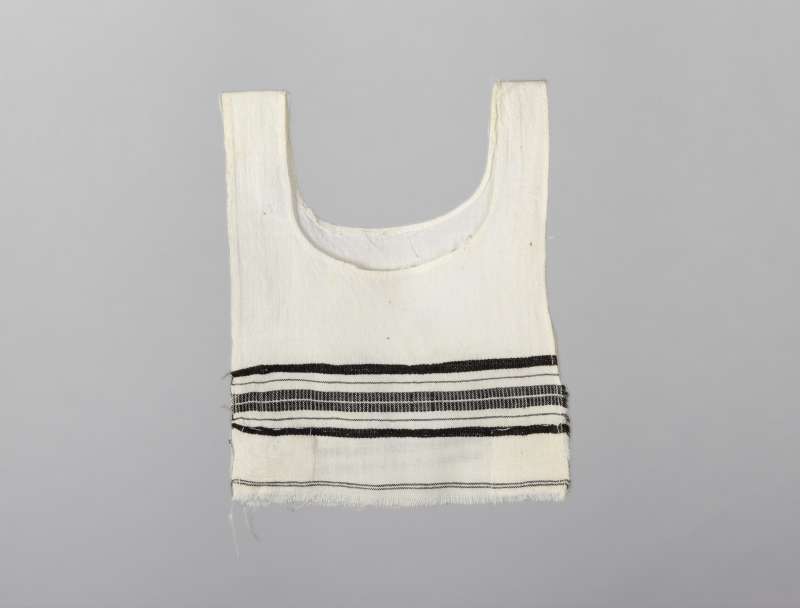This image showcases a handmade, predominantly white crop top that features a unique, detailed design with various stripe patterns. The sleeveless garment is characterized by its low U-shaped neckline and similarly cut back that offers a higher coverage. While the fabric appears somewhat open and frayed at the bottom, adding a rustic, unfinished look, the sides also seem open, further emphasizing its handmade quality. The horizontal stripes vary in color and thickness starting from the bosom: a single black stripe followed by a blue-white stripe, a thin black stripe, a white stripe, then two black stripes interspersed with hints of white. Lower down, the pattern continues with another white stripe, a thin black stripe, a white stripe, a black stripe, a thick white stripe, and finishing off with a trio of thin stripes in black, white, and black. The cloth's texture and patterning bear a resemblance to religious or ceremonial attire, suggesting it might be layered over another garment. The photograph is set against a gray background, further highlighting the intricate details and handmade quality of the top.